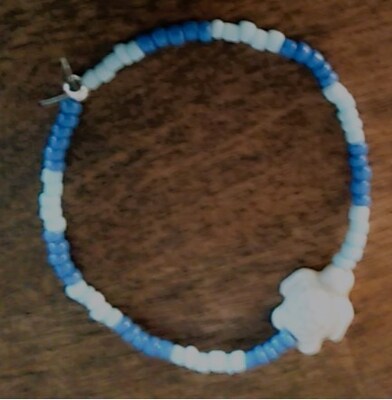This image depicts a small, handmade bracelet placed centrally on a worn black and brown wooden surface. The bracelet, composed of alternating sections of small white and blue plastic beads, appears to be diminutive and delicate. Intricately detailed, it features a larger white bead with ridges—perhaps resembling a star or flower—situated prominently in the middle. In the bottom right corner of the bracelet, a tiny white turtle-like jewel adds a charming touch. Opposite this, on the top left, a small metallic clasp or tie secures the bracelet, preventing it from breaking. The upper blue beads are slightly darker than those at the bottom, adding subtle variation to the piece. Despite the picture being somewhat blurry, the craftsmanship and effort put into creating this bracelet are evident through its intricate design and details.